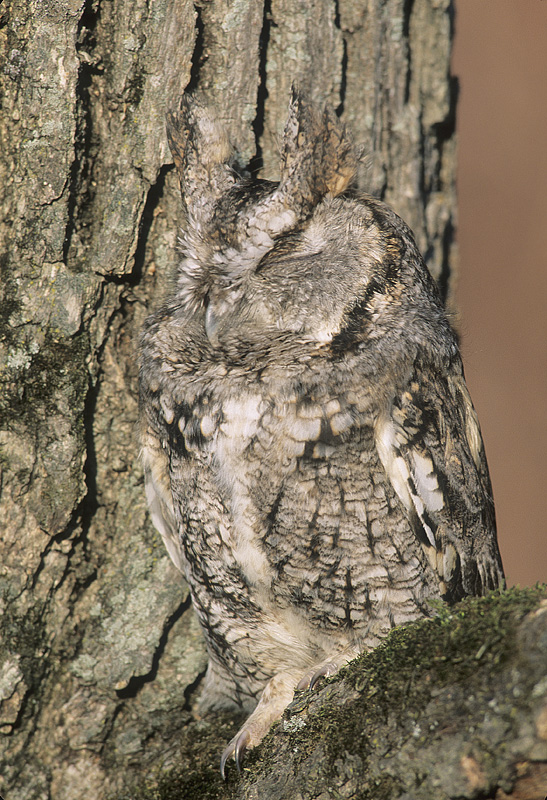The image is an extremely close-up drawing of a grayish-brown tree trunk with rough bark, showing intricate details that indicate an older tree. On a branch decorated with a bit of green moss, an owl is perched while effectively camouflaged, blending almost perfectly into the tree's texture and colors. The owl, with its eyes closed and its prominent ear tufts pointed up, appears to have fallen asleep. Its feathers are patterned in shades of gray, brown, white, tan, and black, mimicking the roughness and tones of the bark, making it nearly indistinguishable from its surroundings. The owl's talons grasp the branch firmly, and its fluffy body is juxtaposed against the tree trunk, highlighted by the subtle background of grayish pink. The meticulous camouflage is so effective that one might overlook the owl at first glance, mistaking it for part of the tree. The background hints at an enclosure, possibly suggesting the setting to be a zoo rather than a wild forest.